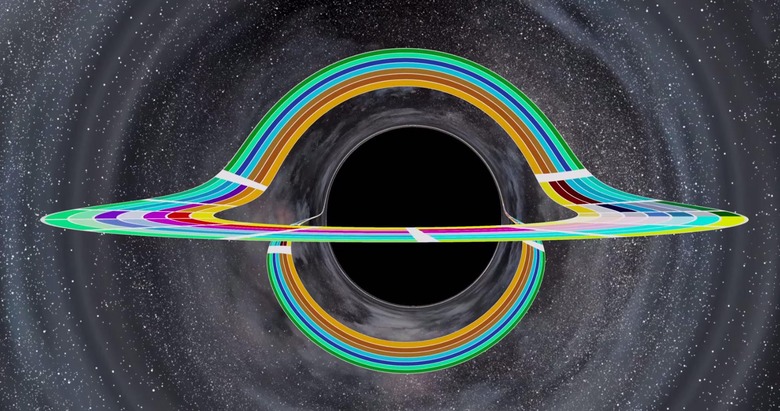This image features a highly detailed and vibrant rendering of an interstellar black hole set against the backdrop of outer space. The black hole itself is centrally positioned, encircled by radial bands of gray and black that shimmer, suggesting the vast, starry expanse of space. A striking feature of the composition is the intricate array of colors forming a semicircular band around the black hole. This band includes shades of blue, yellow, green, orange, red, and additional hues like mint green, forest green, pink, and burgundy. These colors transition seamlessly, creating a visually stunning gradient. Notably, this chromatic semicircle is not perfectly flat; it appears elevated in the top half, as if a frisbee bent upward at the halfway mark, adding a three-dimensional perspective. The lower section of this circle continues beneath, enhancing the intricate, almost sculptural quality of the image. The reflective finish on the colorful band further accentuates the 3D space art style, giving the scene a surreal, yet mesmerizingly beautiful, appearance.